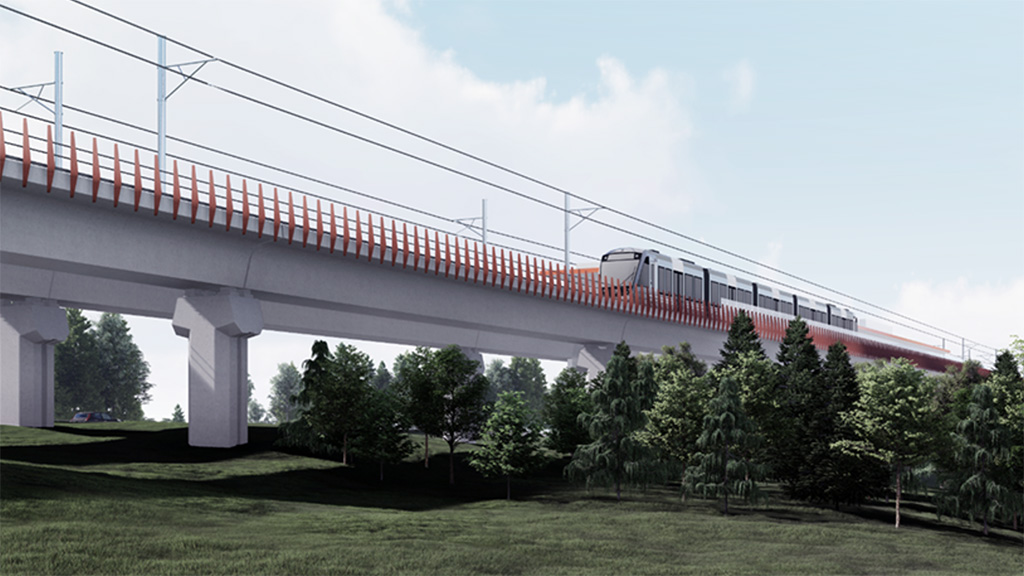In this outdoor scene, an elevated high-speed commuter train is traveling from right to left on a concrete roadway supported by massive cement pillars. The train, comprised of four cars, runs along a track that features distinct orange metal stanchions or bars on the sides. Above the track, power lines are visible. Below, the ground is covered in lush green grass interspersed with various types of trees, including pines. The sky above is adorned with light, wispy clouds, creating a serene backdrop for the modern infrastructure. A white bridge also joins the scene, providing an elegant contrast to the verdant landscape and highlighting the clean, streamlined design of the elevated rail system.